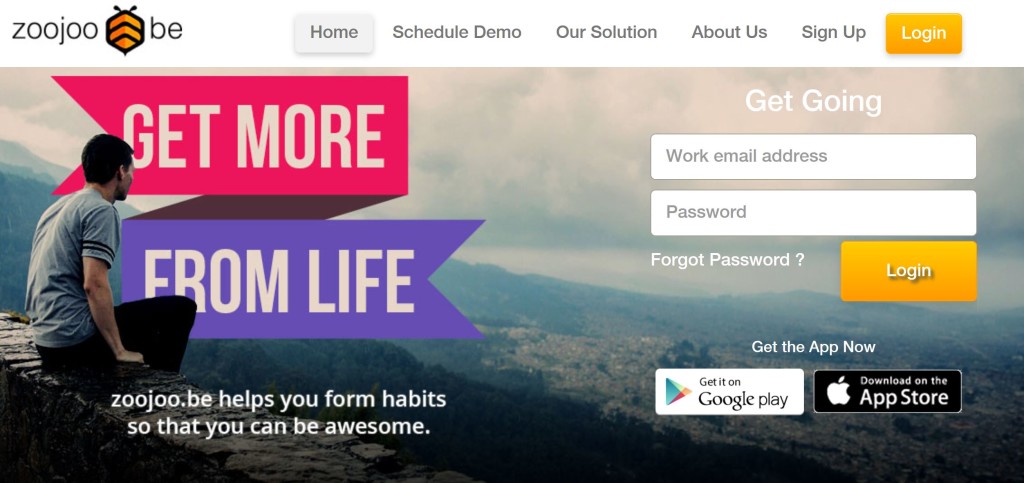The landing page for ZOOJOE.BE features a clean, white background with a navigation bar at the top that includes options such as "Home," "Schedule Demo," "Our Solution," "About Us," "Sign Up," and a prominent yellow "Login" button with white text. 

Below the navigation bar, there is a striking photograph of a man seated on the edge of a wall, overlooking a scenic valley. Superimposed on the image is a ribbon graphic that transitions from pink to purple, bearing the bold, uppercase text "GET MORE FROM LIFE" in white.

Further down, the text "ZOOJOE.BE helps you form habits so you can be awesome" is displayed, emphasizing the platform's mission. To the right of this message, there is a login form with fields for a work email address and password, along with a "Forgot password?" link. The form is topped with a yellow "Login" button with white text.

At the bottom of the page, users are encouraged to download the ZOOJOE.BE app, with Google Play and Apple Store icons provided for easy access. The page is designed with a bright and inviting color palette, featuring splashes of yellow, pink, purple, white, black, gray, green, blue, and red.